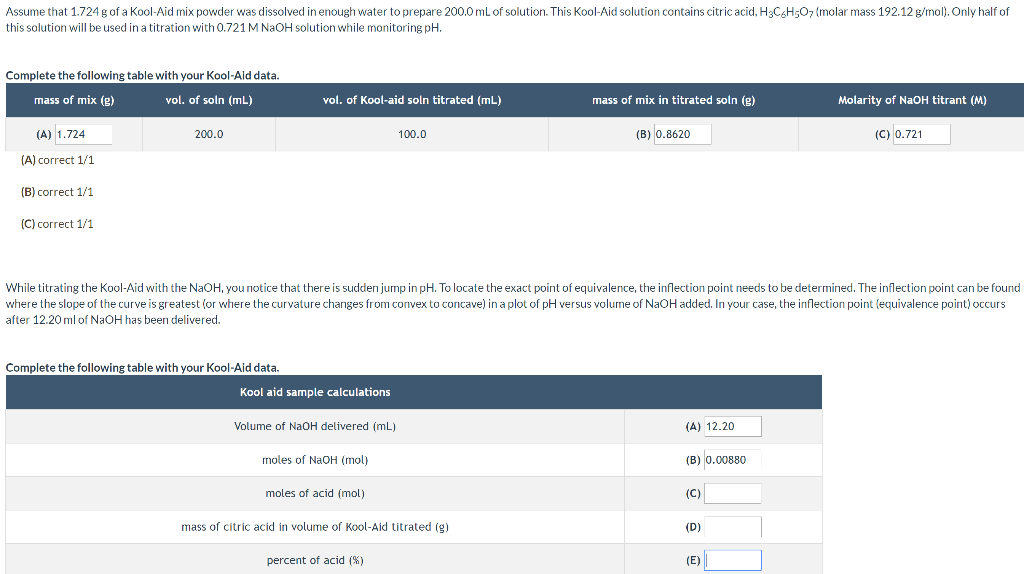In the image, there is both text and two tables. The text, written in dark blue, reads as follows:

"Assume that 1.724 grams of Kool-Aid mix powder was dissolved in enough water to prepare 200 mL of solution. This Kool-Aid solution contains citric acid (H3C6H5O7) with a molecular mass of 192.12 grams per mole. Only half of this solution will be used in a titration with 0.721 M NaOH solution while monitoring pH."

Below the text is the first table titled, "Complete the following table with your Kool-Aid data". It includes the following columns:

1. Mass of mix (A): 1.724 grams (correct).
2. Volume of solution (B): 200 mL (correct).
3. Volume of Kool-Aid solution titrated (C): 100 mL (correct).
4. Mass of mix titrated: 0.8620 grams (correct).
5. Molarity of NaOH titrant: 0.721 M (correct).

Following the table is "Question 2", which states:

"While titrating the Kool-Aid with NaOH, you notice a jump in pH. To locate the exact point of equivalence, the inflection point needs to be determined. The inflection point can be found where the slope of the curve is greatest, or where the curvature changes from convex to concave. In a plot of pH versus the volume of NaOH added, in your case, the inflection point or equivalence point occurs after 12.20 mL of NaOH has been delivered."

The second table is labeled, "Complete the following table with your Kool-Aid sample calculations". The columns in this table are as follows:

1. Volume of NaOH delivered in mL: 12.20.
2. Moles of NaOH: 0.00880 moles (filled).
3. Moles of acid: [empty].
4. Mass of citric acid in volume of Kool-Aid: [empty].
5. Percentage of acid: [empty].